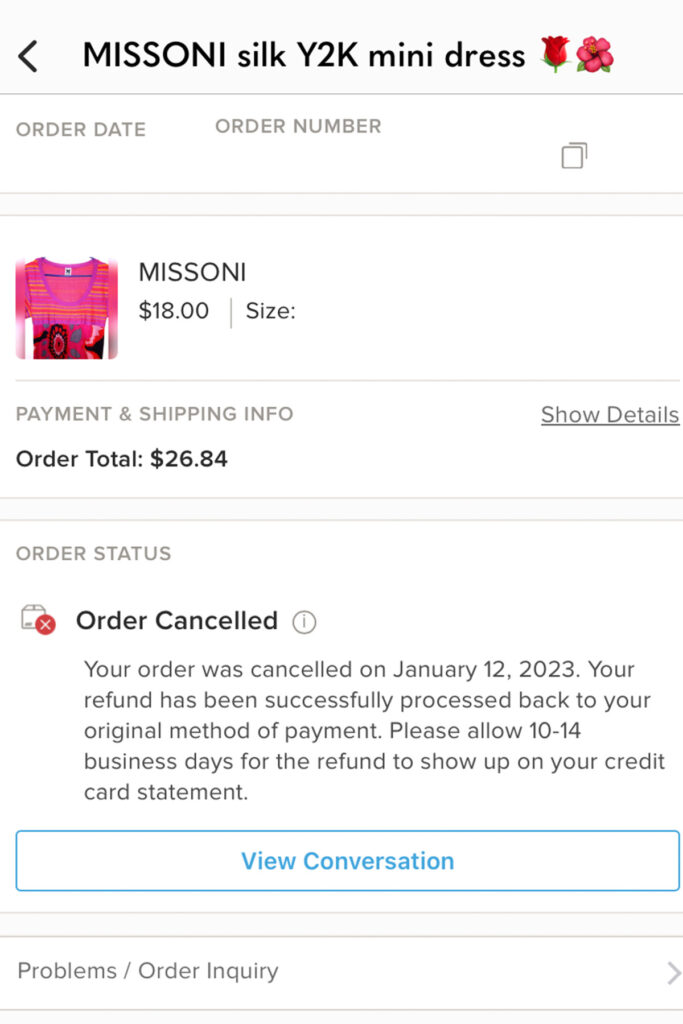**Descriptive Caption for the Image:**

The image appears to be a screenshot from a clothing retail website featuring the details of an order. At the top, in bold, the product name "Missoni Silk Y2K Mini Dress" is displayed, flanked by two flower-like emoji symbols. Beneath this, the order date and order number are provided.

In the center of the image, there is a visual snippet of the mini dress, which is described as having a reddish-purple color with orange floral patterns. Although the complete dress is not visible, it appears to be of mid-length. The dress was priced at $18, but no size information is listed.

Further down, the payment and shipping details are shown. The order total is listed as $26.84, and there's an option to view more detailed information. Moving lower still, the order status section states that the order was canceled, marked with a red X and a small box. An exclamation icon indicates that the order was canceled on January 12th, 2023, with a note that the refund has been processed back to the original payment method, advising 10 to 14 business days for the refund to appear on the credit card statement.

The image also includes a blue box labeled "View Conversation," which seems to outline options for addressing problems or making inquiries about the order. A forward arrow suggests that there may be additional options in a drop-down menu. Notably, a copy button is situated near the order number for easy copying of the order number. The brand name Missoni is mentioned, although it's unclear whether the website itself is Missoni or a different retailer selling Missoni products.